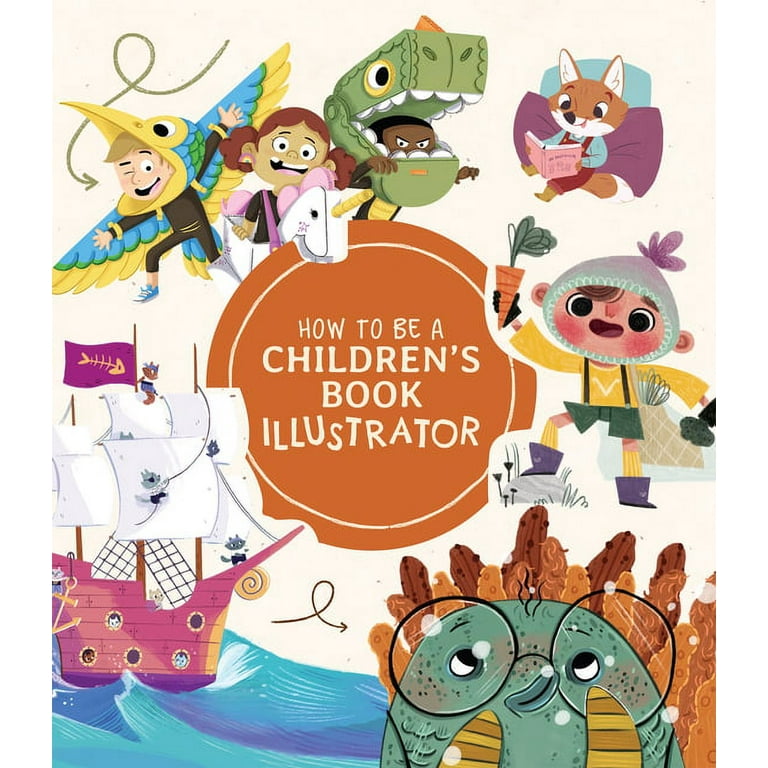The book cover titled "How to be a Children's Book Illustrator" features a whimsical array of characters and scenes designed to spark the imagination. The title is encased in a muted orangey-brown circle at the center of the cover, written in white text. Surrounding this circle, there are charming illustrations you might find in a children's storybook. 

At the top, there's a child dressed in a bird costume with blue wings tipped in yellow and a yellow beak. Next to them are other playful children, including a girl in a unicorn outfit and a boy in a green dinosaur costume. To the right, a cute little fox is engrossed in reading a book. Nearby, a peculiar Martian-like character with a hat can be seen holding a carrot, while another child wears a fish cap.

A small pink pirate ship with big white sails and cats aboard occupies the lower left corner of the cover. Meanwhile, at the bottom right, there's a green, globular creature with gills and glasses, possibly a fish, with a backdrop of brown coral. A mouse is swinging from the pirate ship's sail strings, adding to the lively and adventurous scene. The cover captures the essence of a children's book illustrator, blending fantastical elements with playful and imaginative characters.